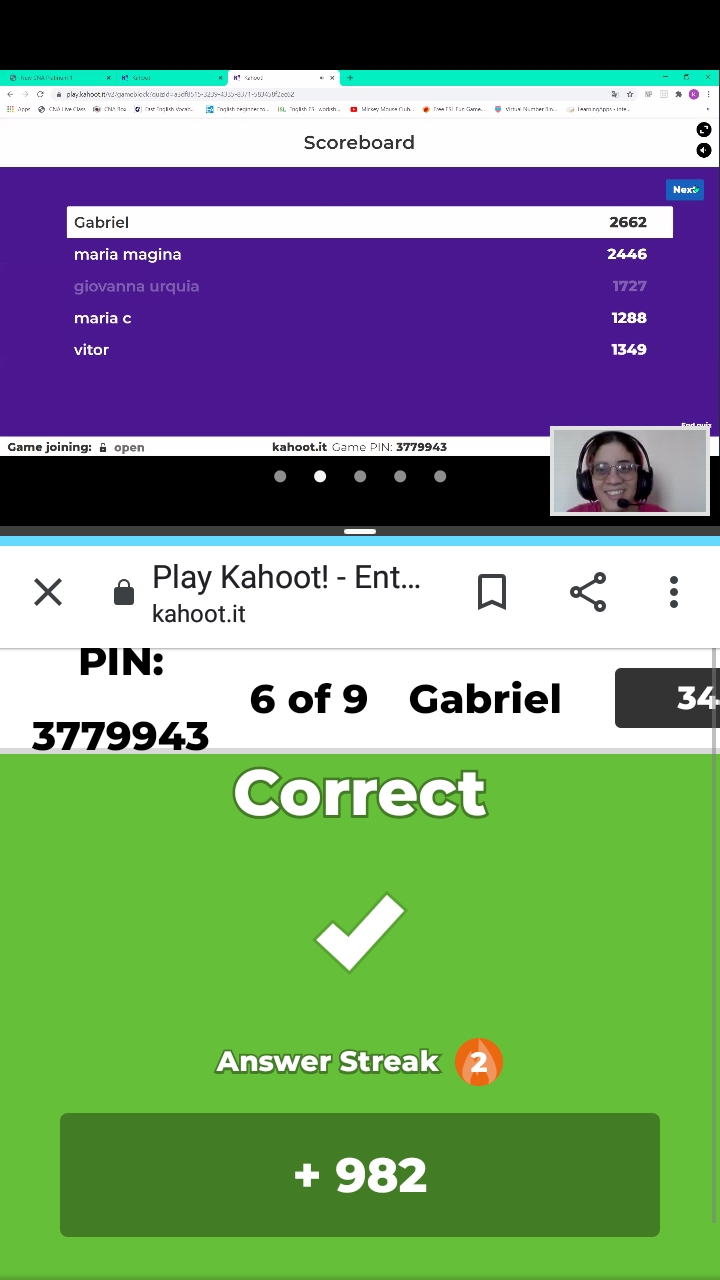This is a color photo of a Zoom session screen capture featuring an online Kahoot game. The screen is split between a leaderboard and the question area of the game interface. At the top, a black stripe displays a scoreboard with "Gabrielle" leading with 2,662 points. Below, the screen shows the game's interaction panel, including four answer squares for participants' choices. The bottom displays "game joining open kahoot.it" and a pin number "3779943". On the left, a green box indicates a "correct" answer with a checkmark, revealing an answer streak of 2 and an additional 982 points for Gabrielle. In the bottom right corner, a smiling woman with a headset is visible against a white background, possibly the teacher or a student. The game is currently on the 6th of 9 questions.